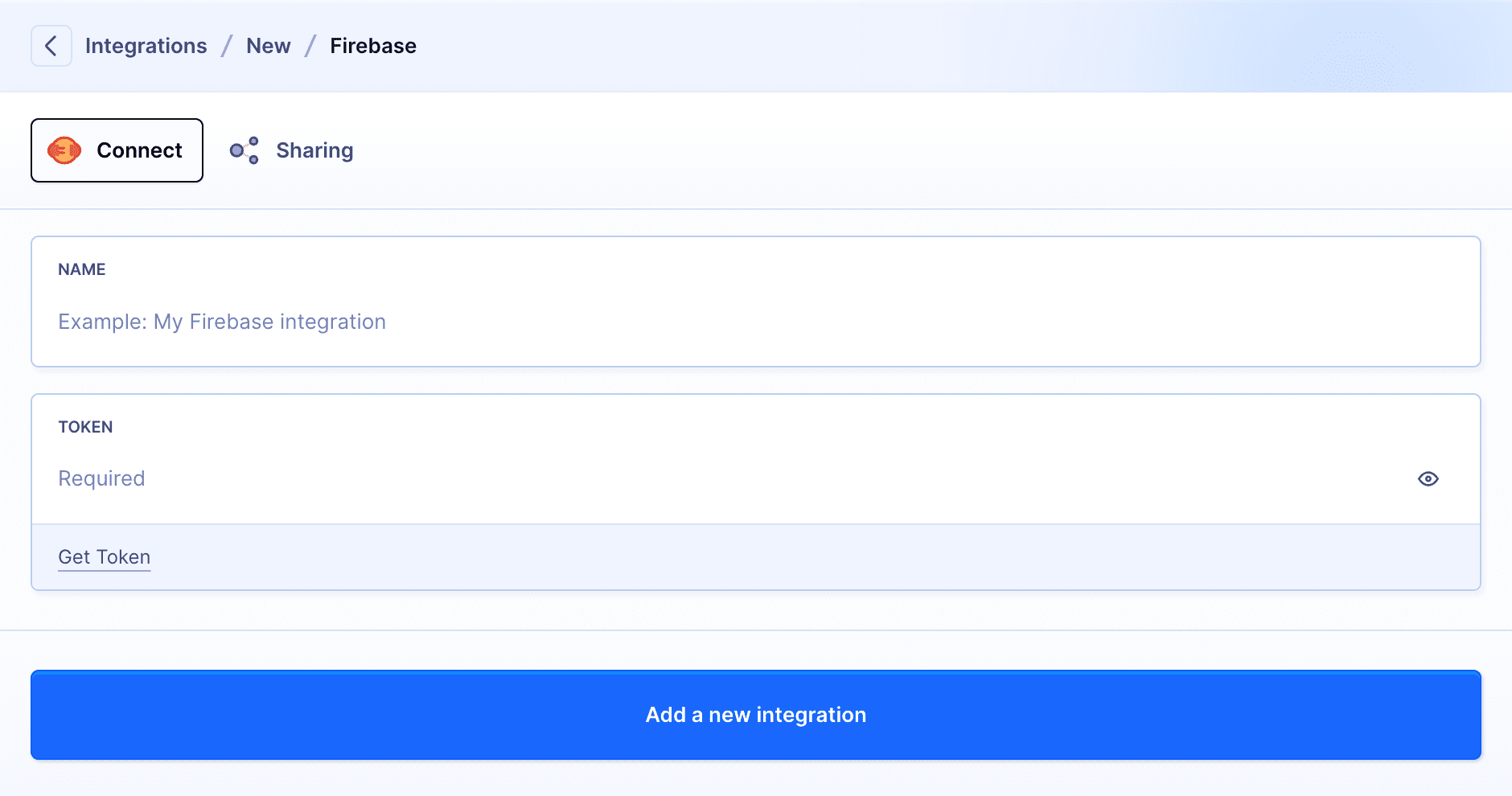Detailed Caption: 

The image showcases a user interface for connecting integrations on a web platform. At the top, the interface has a navigation bar listing "Integrations," "News," and "Firebase," with "Firebase" being highlighted in bold, indicating it's the active tab. Below this, there's a prominent black-bordered button labeled "Connect," adjacent to which sits an icon depicting a plug connecting to an extension cord, symbolizing connectivity.

Further down, a section labeled "Example: My Firebase Integration" appears, indicating a sample or placeholder name for a Firebase connection. Beneath this, there's a text box titled "Token," marked as "required," with an eye icon on the far right side that likely serves as a feature to view or hide the token details. Directly below the token box is a button labeled "Get Token."

At the bottom of the interface, there's a blue, centrally-aligned button with white text reading "Add New Integration Here." This button stands out as one of the few elements with color, signaling its importance in the action flow.

The overall design is set against a white background, with the exception of the "Connect" logo, which features a gradient of orange and red. Navigation arrows are placed to the left, allowing users to go back to previous sections. The interface appears clean and functional, but lacks context on the specific purpose or benefits of the connection beyond the visual indicators and labeled fields.